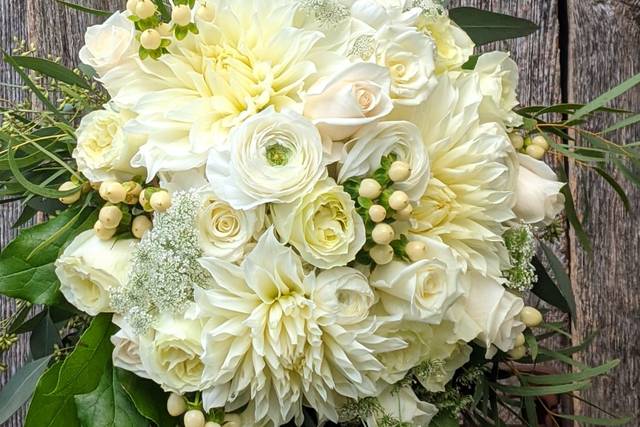The image captures a beautifully arranged bouquet predominantly composed of white roses, both in full bloom and in budding stages, alongside an assortment of other white flowers potentially including Queen Anne's Lace or Baby's Breath, interspersed with delicate white berries. The flowers are accompanied by lush green leaves that add depth and texture to the arrangement. This lovely bouquet is placed on a weathered, unvarnished wooden surface, likely outdoors on a rustic table or deck, as evidenced by the vertical grain of the wood, which suggests a natural, weather-exposed environment. The bouquet exudes elegance and charm, reminiscent of a bridal accessory or a cherished arrangement at a joyous outdoor gathering.